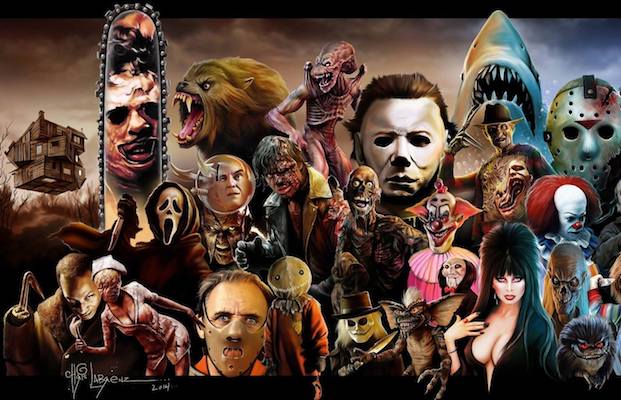The image is a detailed and elaborate collage of iconic horror movie characters set against a dark, ominous, and somewhat stormy gray sky. The menacing sky peeks through the gaps between the densely placed images. Dominating the collage are various infamous villains: Leatherface framed by the edges of a chainsaw, multiple masked Mike Myers, the formidable Jaws shark emerging with its mouth wide open, Freddy Krueger with his razor glove poised, Pennywise the Clown, and Elvira, Mistress of the Dark, with her signature black outfit and spiky hair.

Additional figures include Hannibal Lecter in his recognizable mask, the Phantom of the Opera with his white mask and auburn hair, and Jason Voorhees with his hockey mask. A creepy clown (likely from "It") is positioned near Elvira. The collage also features an array of lesser-known ghouls, such as a nurse with a distorted face, a creature with a bag over its head, the Cryptkeeper, and a character with a hook hand. There are also gremlins, a zombie, a sinister little puppet from "Saw," and the masked figure from "I Know What You Did Last Summer." Above, the top left hosts a house from "The Wizard of Oz," seemingly floating amid the stormy backdrop. An alien and a werewolf add to the eerie ensemble. The image is bordered in black on both the top and bottom, giving it a framed, compact feel, while a signature in white marks the bottom left corner.